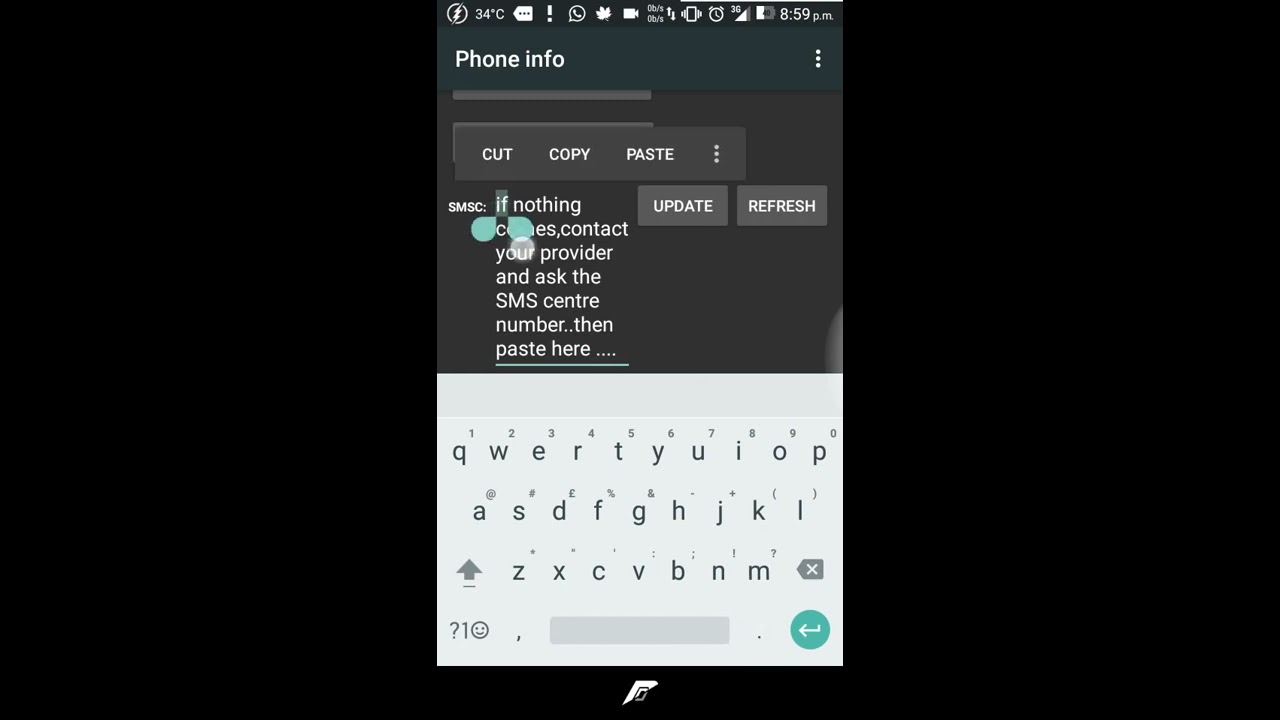Detailed Caption:

This is a detailed screenshot from a mobile or tablet device that is currently charging. The device screen shows a temperature of 34 degrees Celsius and displays multiple notifications. Among these notifications are an old price tag icon and an exclamation point symbol, accompanied by the WhatsApp icon and a maple leaf. Additionally, a webcam icon indicates that there is no active upload or download activity.

The device is set to vibrate mode and an alarm is scheduled. The network connection is 3G with a signal strength of three out of four bars. The battery level is at 40%, and the time displayed is 8:59 PM, though the charge icon to the left does not correspond to the battery indicator.

The screen also shows detailed phone information and a context menu, represented by three vertical dots on the right. This menu is currently active and offers options such as cut, copy, and paste, along with more options accessible through additional three vertical dots. Options under this extended menu include "update" and "refresh." An instructional message reads: "SMSC: If nothing comes, contact your provider and ask for the SMS center number, then paste here." The word "if" is highlighted with pale green teardrops, suggesting the user is interacting with this text.

Below this text entry field, the user's lowercase keyboard is visible, implying that they are possibly in the process of updating their phone settings.